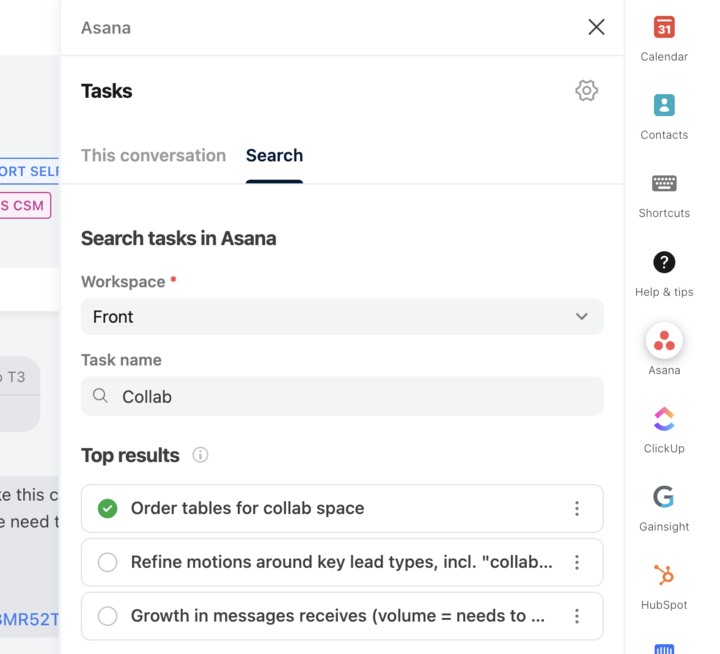This image is a screenshot taken from a computer, iPad, or cell phone, displaying the Asana application interface. At the top of the screen, the word "Asana" is prominently displayed, followed by an "X" button on the right for closing the interface. Below, a bold black header labeled "Tasks" is visible, right above a subtitle that reads "This Conversation."

Further down, there's a search area with a black underline labeled "Search," and immediately below it, the text "Search Tasks in Asana" is shown. Additionally, "Workspace" and a drop-down arrow for selecting "Front" or other options are present. The search bar contains the term "Collab" (C-O-L-L-A-B).

Scrolling down the interface reveals top search results including an item marked by a green circle with a white checkmark, labeled "Order Tables for Collab Space." Below this are several unchecked items.

On the right-hand side, a vertical panel contains clickable icons for features such as Calendar, Contacts, Shortcuts, and Help and Tips. The panel also lists integrations or related applications including Asana, ClickUp, GainSite, and HubSpot.